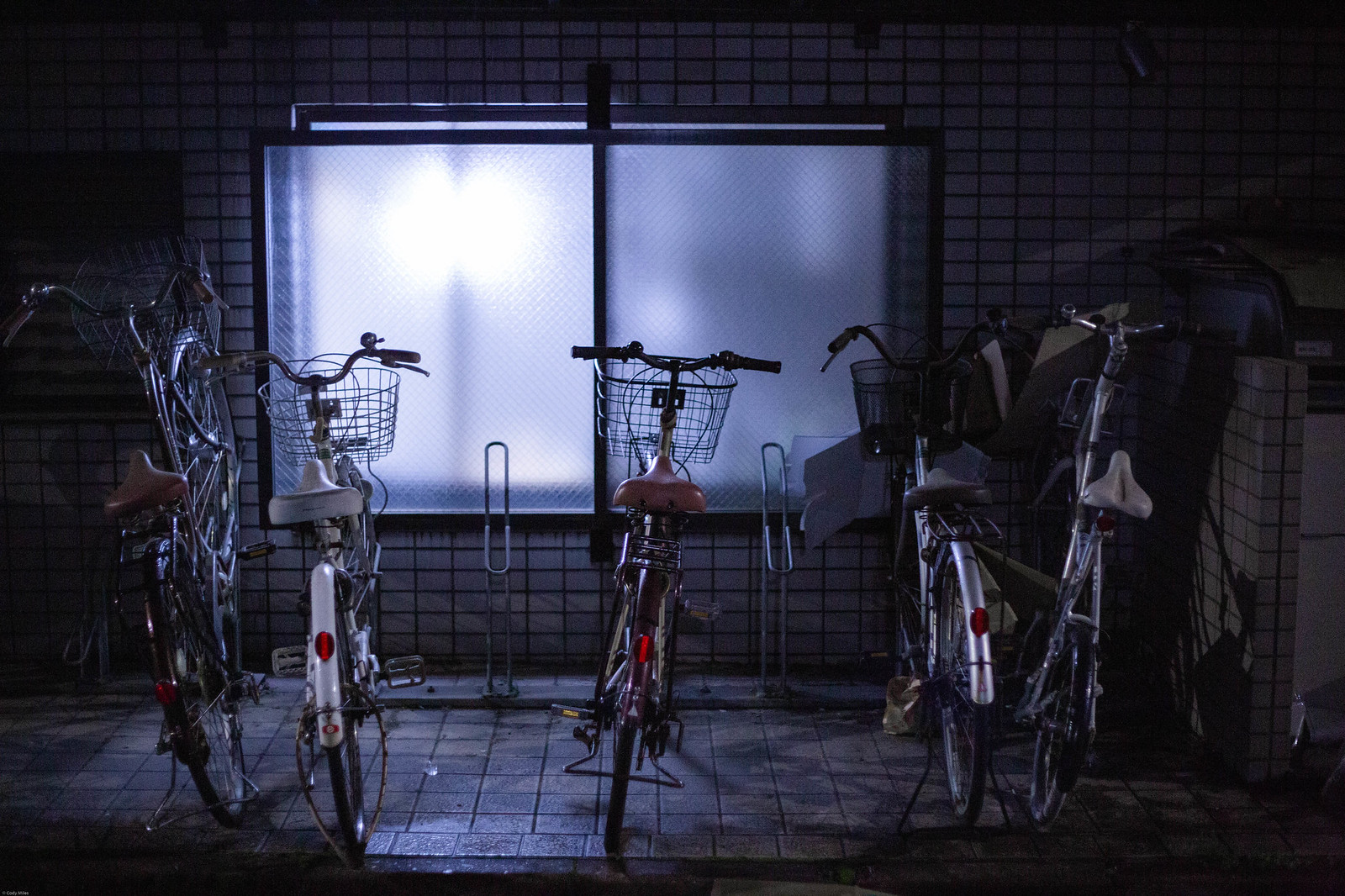This photograph, likely taken at night outside a building, captures five bicycles parked in a row. The backdrop consists of a white-tiled wall made of small bricks, with black or extremely dark gray mortar. Dominating the center of the image is a double window with frosted glass that permits diffused light to shine through, revealing no interior details. The window also features a mesh layer for added safety. The bikes are neatly arranged in a metal bike rack that can accommodate up to seven bicycles, positioned on a tiled sidewalk. 

Starting from the left, the first bike, with a black frame and brown seat, leans slightly as if planted on the bike rack. Following it, the second bike has a white frame and white seat, secured with a distinctive cable bike lock on the rear tire. The third bike features a black frame with a brown seat, while the fourth sports a black frame and black seat. The fifth bike, positioned farthest to the right, also has a black frame paired with a white seat. Each bike is equipped with wire baskets at the front, and some even have bells. The seats exhibit a pattern with colors alternating among brown, white, and black.

The bikes vary slightly in color, but all share common safety features like red reflectors on the rear. The rear wheel covers change colors from dark brown on the leftmost bike to white, dark brown, silver, and black on subsequent bikes. The overall scene, with the shadowy ambiance and strategic lighting from the window, evokes an atmosphere typically found in urban settings, possibly Japan.